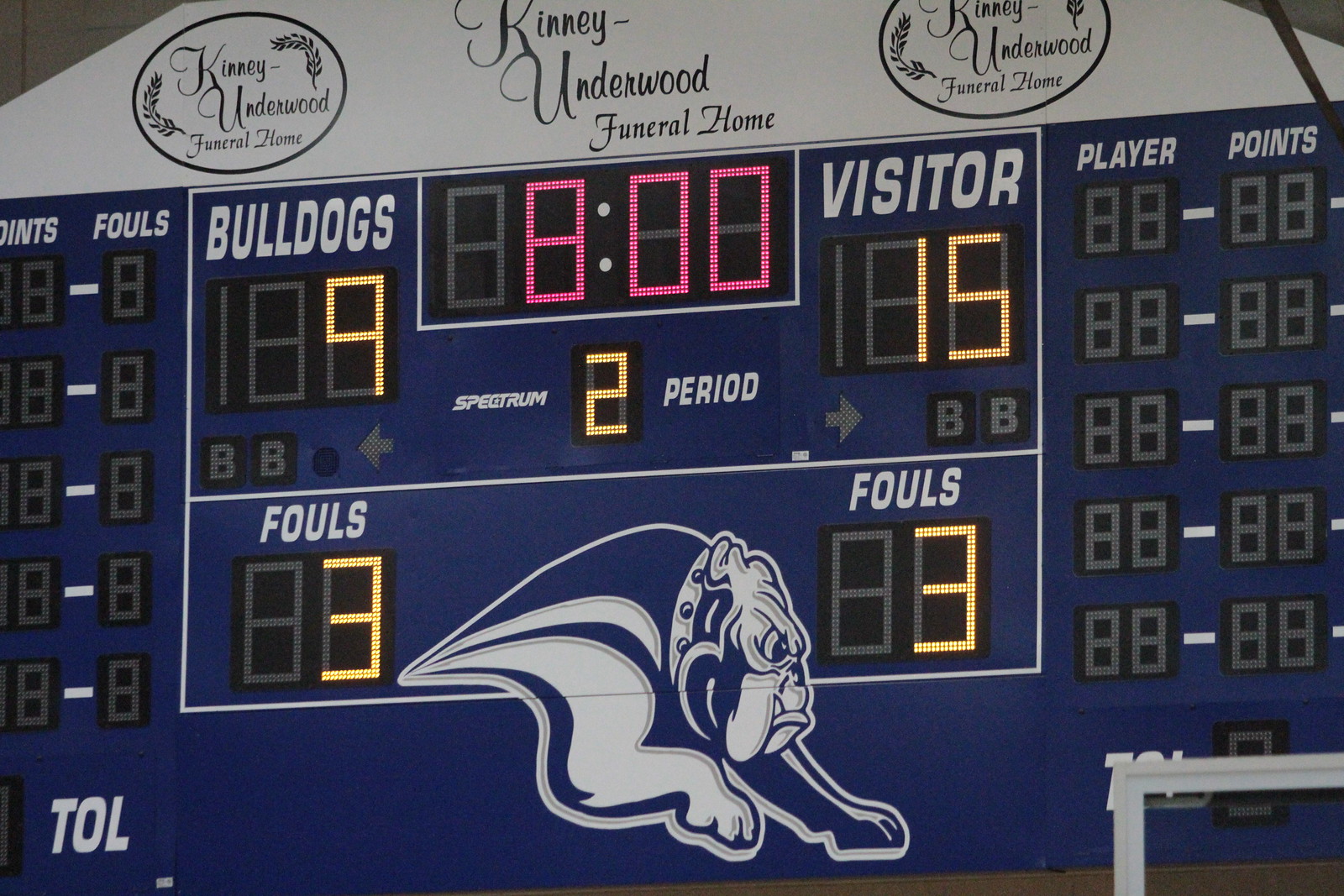The image is a detailed photograph of a gymnasium's digital scoreboard. The scoreboard is predominantly blue and is topped with an advertisement for "Kenny Underwood Funeral Home," displayed on a white arched area with black font. This name appears again in black-framed circles on either side of the top. Centrally located, the scoreboard shows a time of 8:00 in pink LED, with other critical information in yellow LED lights.

On the left side of the scoreboard, the title "Bulldogs" is displayed, with a digital section underneath showing a score of 9 points and 3 fouls. Similarly, on the right side, the title "Visitors" is shown, with a digital section indicating 15 points and 3 fouls. At the bottom of the scoreboard, there are additional titles reading "Fouls" with corresponding digital signs underneath for each team. An illustration of a Bulldog mascot is present between the Bulldogs' and Visitors' foul indicators, adding a touch of school spirit to the otherwise functional design. The detailed and well-organized layout suggests a high level of school pride and sponsorship by the Kenny Underwood Funeral Home.